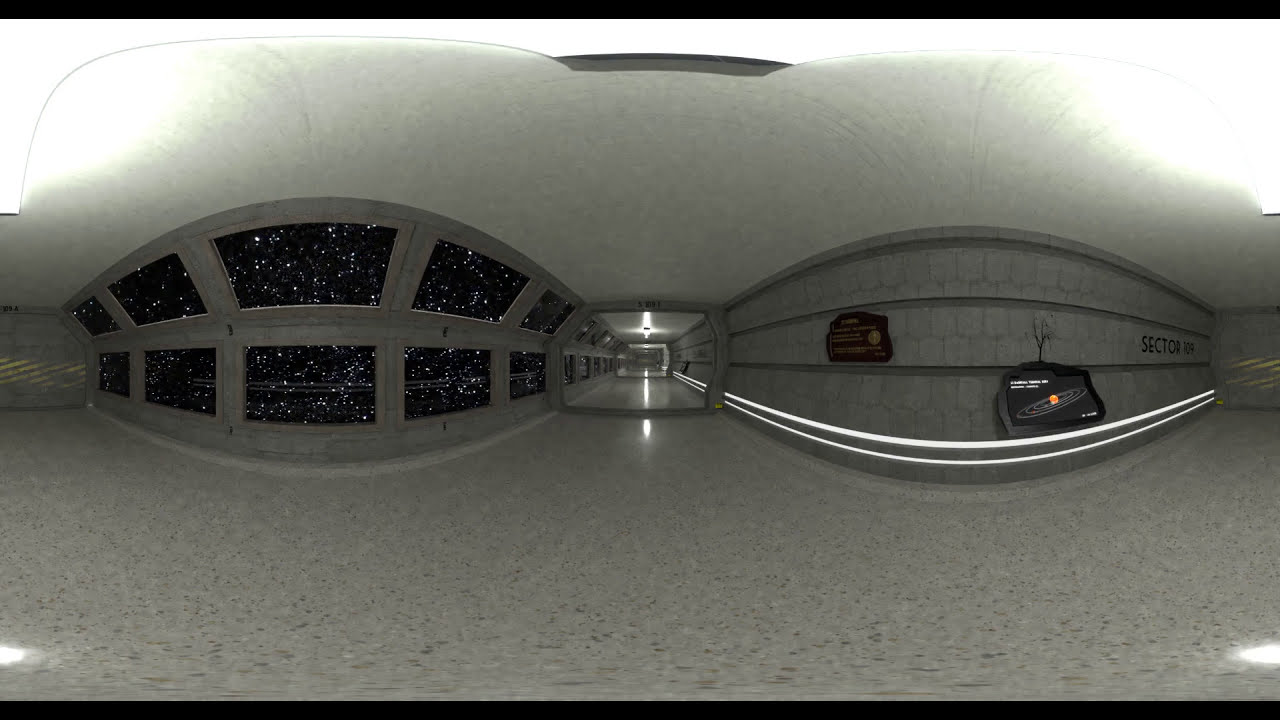The image depicts a fisheye view of a vast and distorted interior of a public planetarium designed to educate visitors about space. The surroundings are predominantly gray, with an arched ceiling and walls creating an expansive yet enclosed atmosphere. The left side features multiple segments of a black starscape, divided into numerous boxes with gray frames, showcasing twinkling starlight that stretches extensively. In contrast, the right side is characterized by gray paneling marked with the label "Sector 309," accompanied by an illustration of a ringed planet. Notably, there are no people present in the photo, and the shiny, reflective floor appears to be made of marble.

The wide hallway, illuminated from the top left and right, features long, straight corridors leading to what seems like glass enclosures or walkways at the ends. Amidst the central area, a glass square stands, its precise function ambiguous due to the distortion—is it a mirror or a door? On one wall, shelves host a picture and a TV, while the opposite wall is adorned with black squares dotted with white, resembling stars in the night sky.